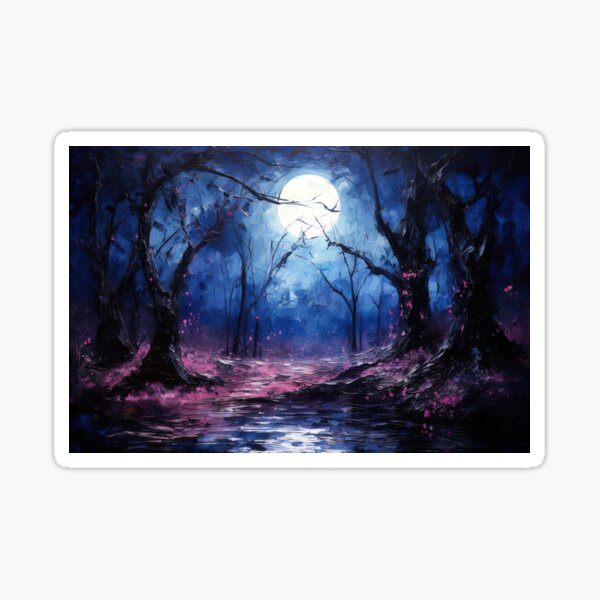This image depicts a hauntingly atmospheric painting showcasing a spooky nighttime forest scene. Dominated by a bright, full moon centered at the top, the moonlight cascades down, creating eerie silhouettes of four large, leafless trees with black, oak-style trunks and spindly branches. These trees frame a narrow pathway that meanders through the forest, leading the viewer's eye deeper into the mist-laden, surreal landscape. The ground and distant areas are tinted with purples and dark blues, with some pinkish-hued mist or foliage around the trees on the left, adding to the fantastical feel of the scene. The entire composition, with its visible brush strokes and almost melting appearance, evokes a sense of mystery and foreboding, making it an ideal backdrop for a spooky tale or a Halloween setting. The painting is set against a light gray background, bordered in white, enhancing its dream-like quality.